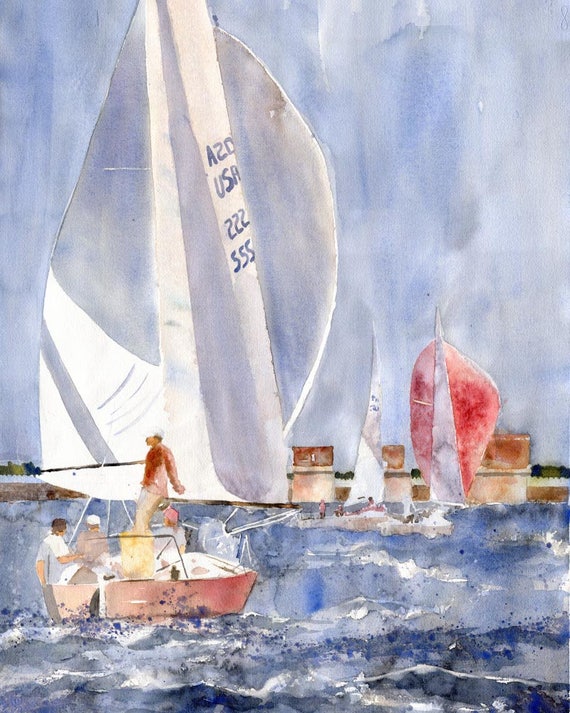This watercolor painting depicts a lively ocean scene characterized by choppy, royal and navy blue waters with prominent white-tipped waves. Central to the image is a light coral-colored, almost rectangular fishing boat carrying four men. The boat has a strikingly large white sail, held up by a mast or tripod structure, adorned with blue text: "A20 USA 222555." Surrounding the primary vessel, the background features more boats, blurred to suggest distance, one with a white sail and another with a red-and-white sail. Hints of a lightly clouded, yet predominantly blue sky further emphasize the serene yet dynamic nature of the scene.